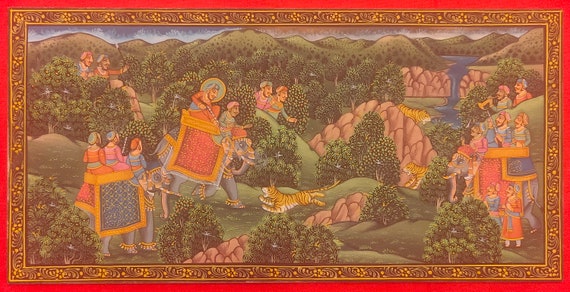This image depicts an elaborate and detailed tapestry or painting with a red-bordered frame and an ornate, gold fleur-de-lis patterned inner border. The central scene, characterized by its lush greenery and vibrant colors, shows people riding elephants through a dense forest with rolling hills and rock formations. The elephants, adorned with textured cloths in hues of red, blue, and gold, carry groups of two to three people each. Some figures appear to be carrying spears, and one might be playing a trumpet, contributing to an almost festive atmosphere. A river fed by a waterfall runs through the background, adding to the serene, lush landscape. Adding an element of wildlife, a tiger and potentially some cubs are also present among the bushes, as well as a dog with a yellow coat barking at the elephants in the bottom left corner. The scene is rich in detail, with additional features like a gray sky peeking through tree-covered mountains, contributing to the impression that this is a historic or possibly Biblical depiction.